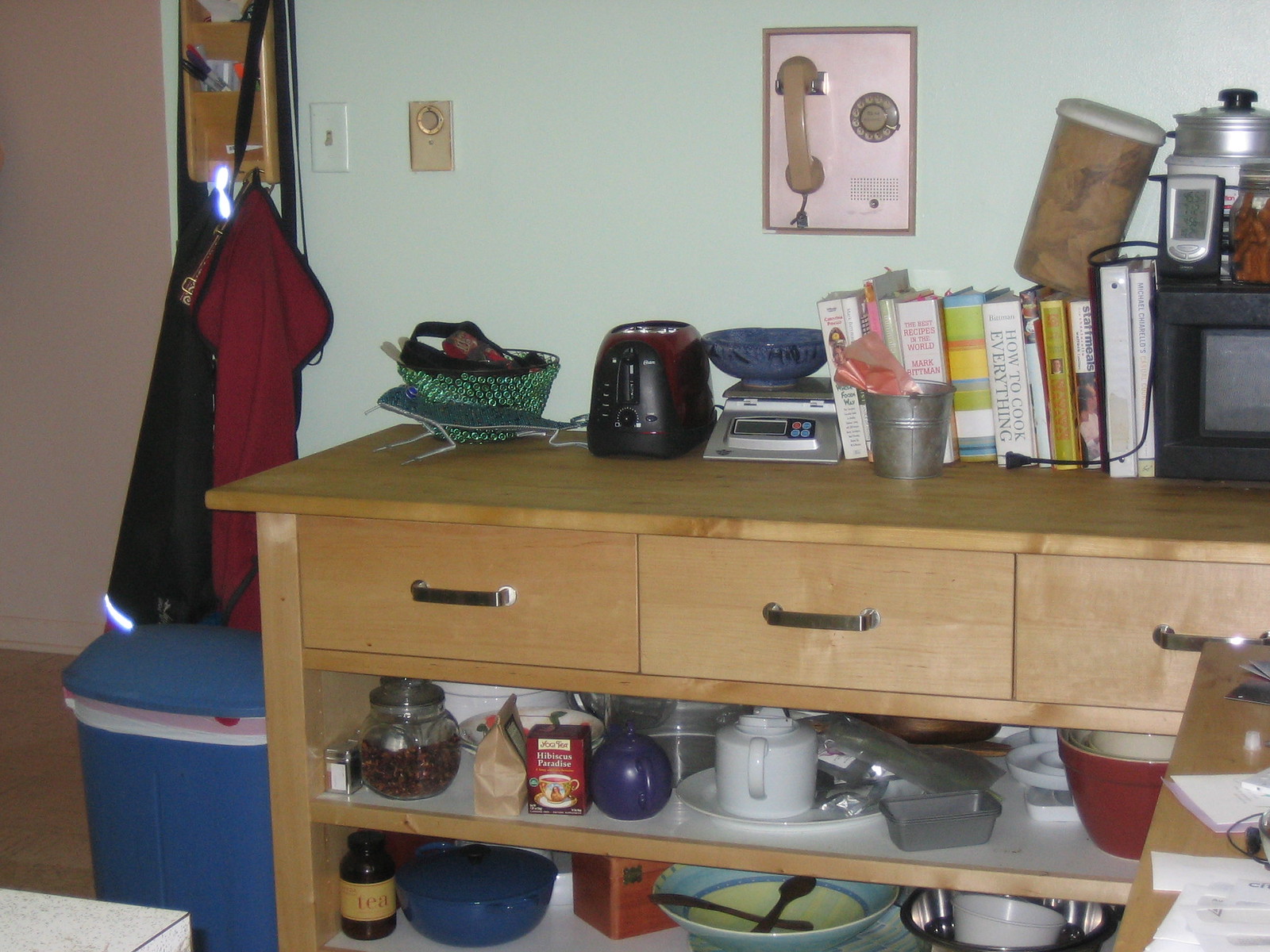This image captures the interior of a cluttered, retro-style kitchen, photographed in landscape orientation. The kitchen features a mint green wall that is adorned with a vintage rotary telephone. The telephone's handle is a tan taupe color, and it is mounted within a square frame that has a pink background. Directly below the phone, there is a small tabletop collection consisting of various books, a microwave, a toaster oven, and a green fruit bowl. These items rest atop a light wooden cabinet with visible grain and drawers.

Additionally, the lower portion of the image reveals a disorganized assortment of dishes stored beneath the wooden casing. On the left side of the scene, a blue trash bin lined with a white trash bag stands next to the cabinet. Above the bin, two aprons—one red and one black—hang neatly, adding to the everyday, lived-in aesthetic of the kitchen. The overall composition of the photograph highlights a space that is both functional and nostalgically charming, with a blend of modern necessities and vintage accents.